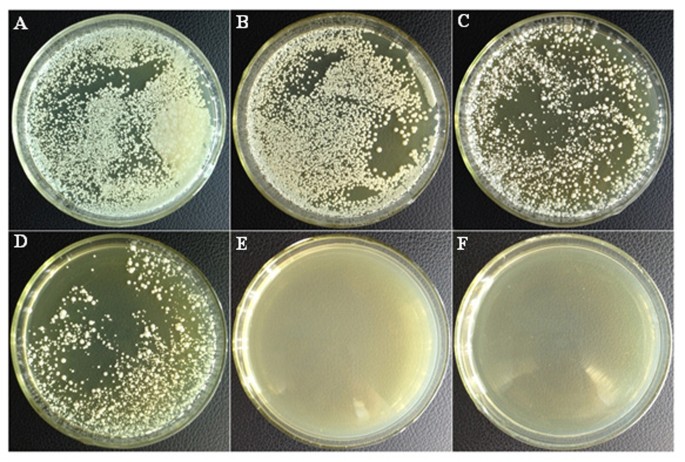This image depicts six Petri dishes arranged in two rows of three, atop a black leather-like surface. Each Petri dish is labeled sequentially with white text: A, B, C, D, E, and F. The dishes are occupied by varying quantities of a whitish, possibly yeast-like or bacterial growth, which appears as a white, fuzzy substance. Petri dish A, located at the top left, contains the most substantial growth, which progressively decreases through dishes B and C. Dish D, at the bottom left, has slightly less growth than C. The growth further diminishes in dish E, and by dish F there is no visible growth at all. This arrangement visually illustrates a gradation in the proliferation of the biological substance from A to F.